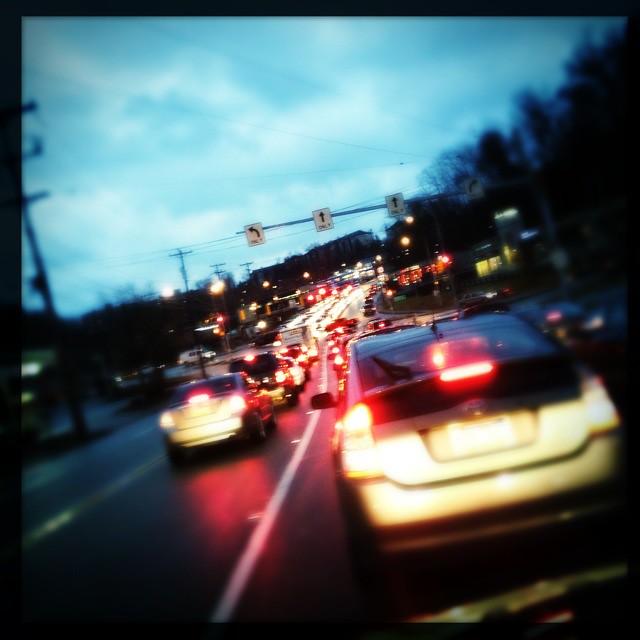This photograph captures the view from within a car, looking out through the windshield at a line of vehicles ahead as it sits in what appears to be heavy traffic during dusk. The streetlights are already illuminated, casting a soft glow over the scene, and all the cars have their headlights on. The most immediate vehicle in the foreground is a silver Toyota Prius. Lining the right side of the roadway are trees, their dark silhouettes contrasting against the gradually dimming sky. An overhead traffic sign is visible above, displaying directions for the lanes: left turn, straight, and right turn only. The overall scene is tinged with the hues of early evening, as both natural and artificial lights blend to create a quintessential rush-hour moment.